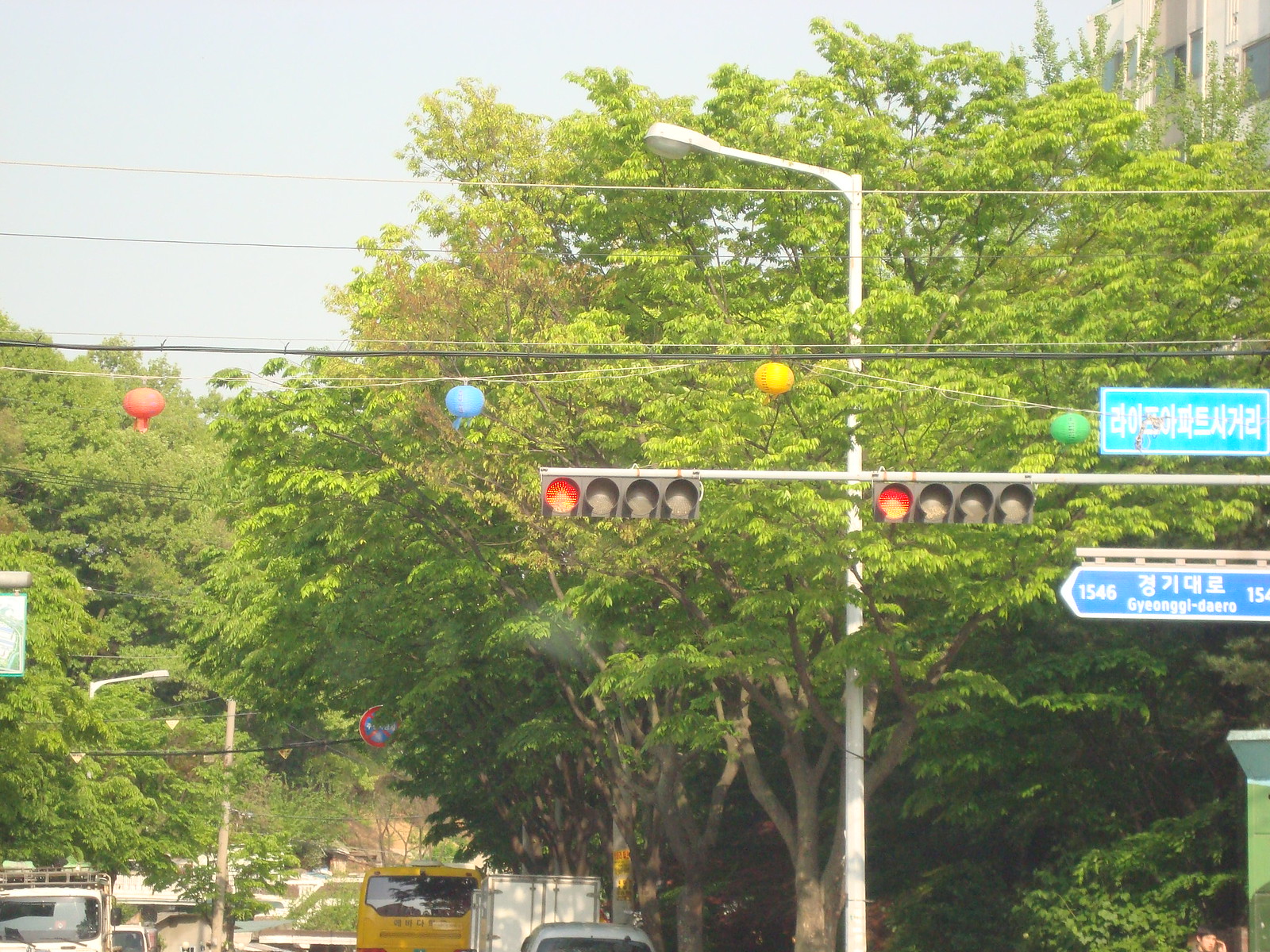The image depicts an outdoor urban setting featuring a prominent stoplight that currently shows red. The stoplight, mounted on a white pole, has four lights and is flanked by power lines overhead. On these power lines are four hanging colored balls in sequence: red, blue, yellow, and green. In the background stands a streetlight in front of a large, lush green tree. The scene also includes multiple vehicles visible at the bottom, including a distinctive yellow bus with a glass back. Towards the right side of the image, blue street signs and another sign with the number "1546" can be seen. Some of these signs, as well as additional text on the image, are written in a foreign language, likely Asian. The overall setting appears to be taken on a bright, sunny day.